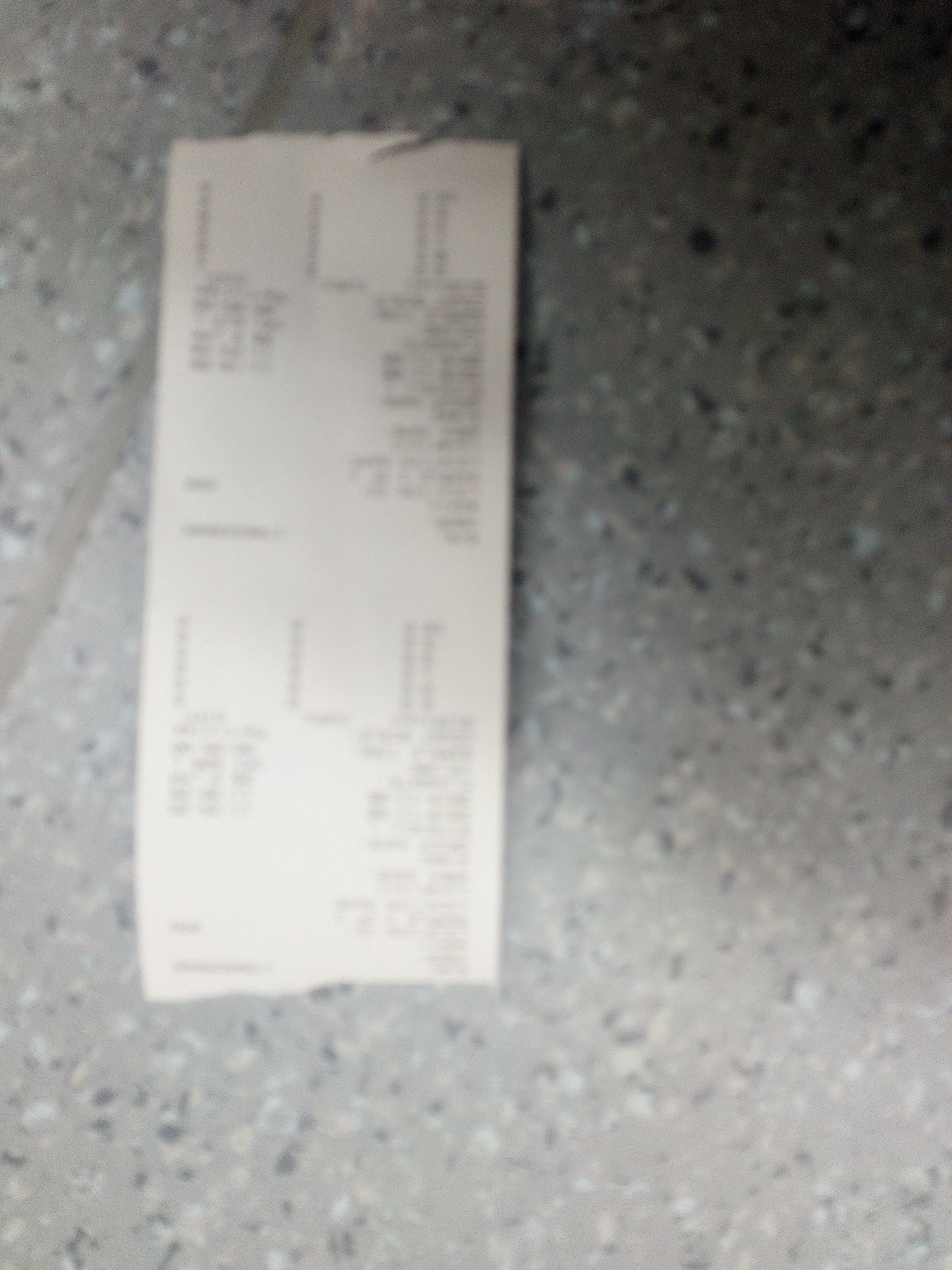This image is a very blurry close-up of what appears to be a small, off-white receipt, positioned slightly to the center left. The background looks like a speckled surface, possibly a countertop or an epoxy-finished floor, featuring a mix of gray, dark gray, cream, and specks of white and bluish tones. This surface also has a noticeable line running from the middle of the picture towards the top left corner, likely a piece of caulking. The receipt, possibly upside down, seems to be connected at the top by a metal ring and features numerous illegible printed words and numbers, similar to typical receipt formatting. The overall image is heavily blurred, rendering all the text on the receipt unreadable and obscuring finer details.